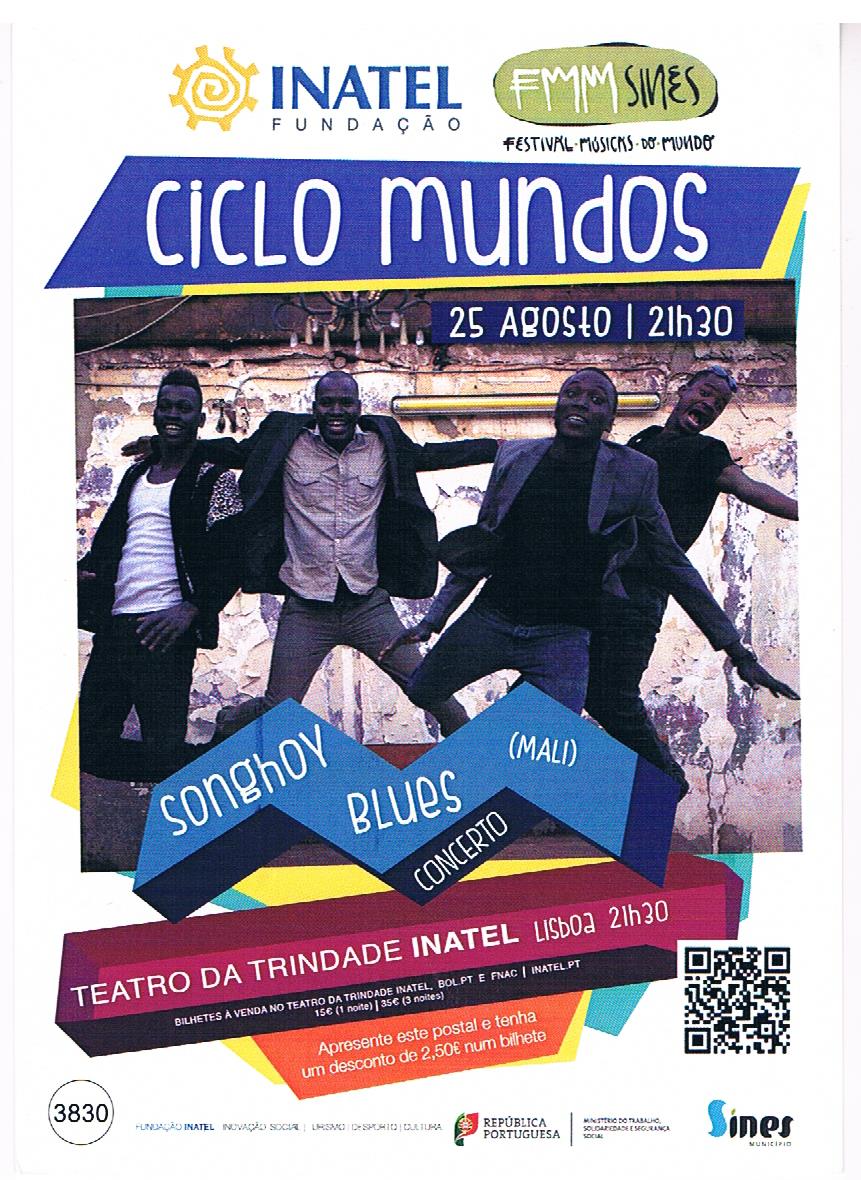The image is a colorful advertisement poster for a music festival named "Ciclo Mundos," organized by Inatel Fundacao. At the top, the Inatel Fundacao logo, featuring a circular spiral with square points, is displayed next to the festival name. The text, "Republica Portuguesa," suggests it takes place in Portugal. Highlighted in various vibrant hues such as blue, red, yellow, orange, and pink, the central image features four African men, possibly musicians, dressed in assorted outfits including a white tank top, an open shirt, and a suit jacket. They are lively and animated, engaging with the camera. The event, which is a "Songhoi Blues Mali Concerto," is scheduled for August 25th at the Teatro de Trinidad Inatel. Additional details, like a green circle with "FMM" and various colored shapes and text boxes in foreign languages, add to the design complexity. Promotional elements, including a barcode and a circular "3830" at the bottom, alongside advertising text, complete the vivid layout.